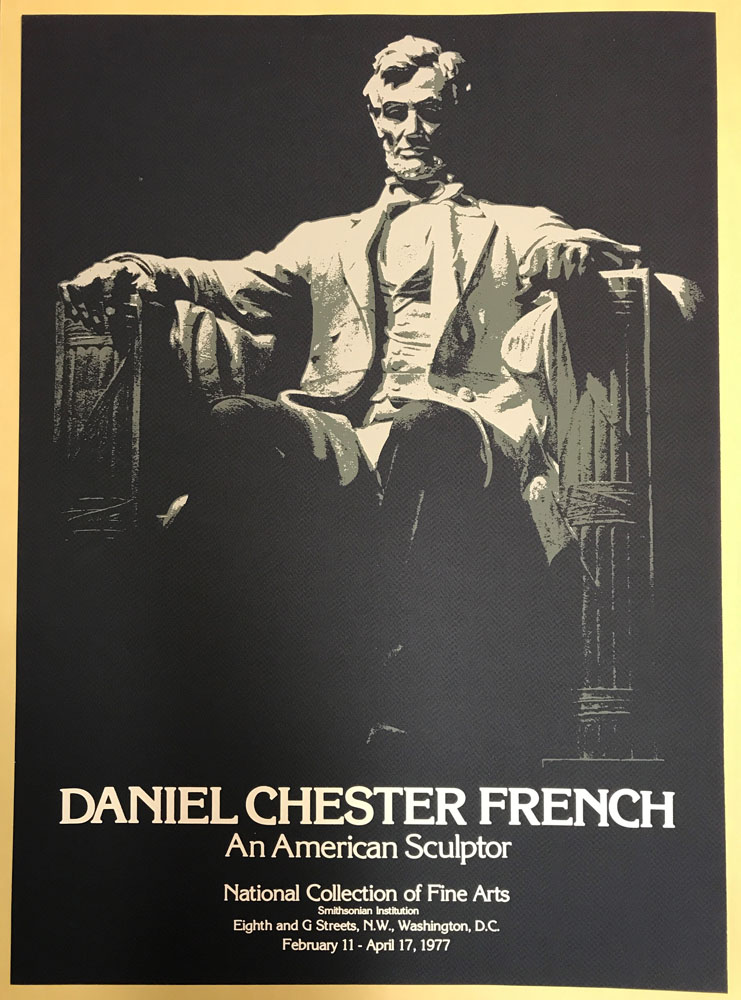This black-and-white poster advertises an art exhibition at the National Collection of Fine Arts, showcasing the work of American sculptor Daniel Chester French. The main feature of the poster is an image of French's iconic sculpture of Abraham Lincoln as seen in the Lincoln Memorial. Lincoln is depicted seated in a high-backed, high-column armchair, radiating a stark contrast against the black background. Above the image, there is a narrow yellow border framing the poster, which shows slight warping, particularly on the right side. Below the sculpture, in large bold white uppercase letters, the text reads "DANIEL CHESTER FRENCH." Underneath, in smaller white text, it states "An American Sculptor." Further down, the text provides details about the exhibition location and dates: "National Collection of Fine Arts, 8th and G Streets, NW, Washington DC," followed by the exhibition dates, "February 11th - April 17th, 1977."